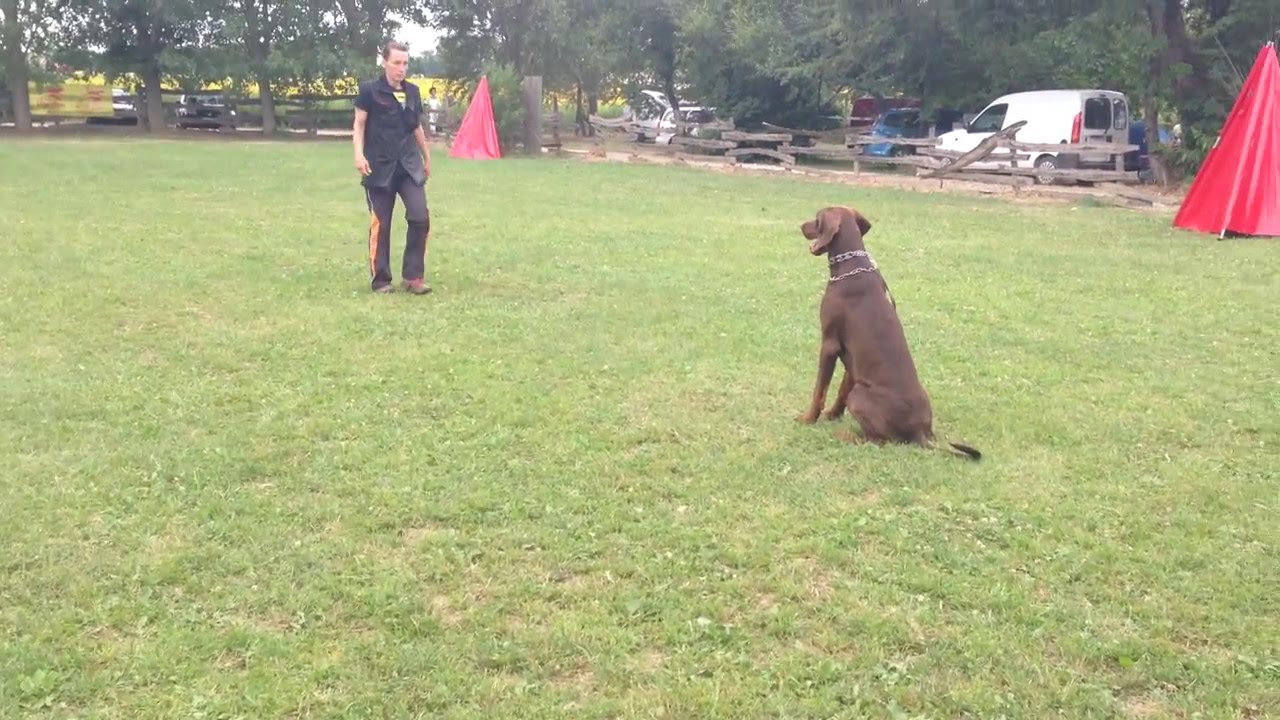In this vibrant outdoor park setting on a sunny day, a white man dressed in a black outfit—comprising a button-up shirt and pants with an orange stripe down the side—stands on a lush green patch of grass. About 20 feet away from him is a chocolate-colored Labrador Retriever, which is seated and wearing a collar, suggesting a training exercise or moment of interaction. The scene is framed by several background elements: a wooden fence extending across the area, a collection of parked cars including a white minivan and a mix of blue and white vehicles, and two distinct red tent-like structures, one directly behind the man and another visible in the top right corner. The image also captures the serene atmosphere with clear skies, scattered trees, and an open grassy expanse, creating a picturesque and tranquil park environment.